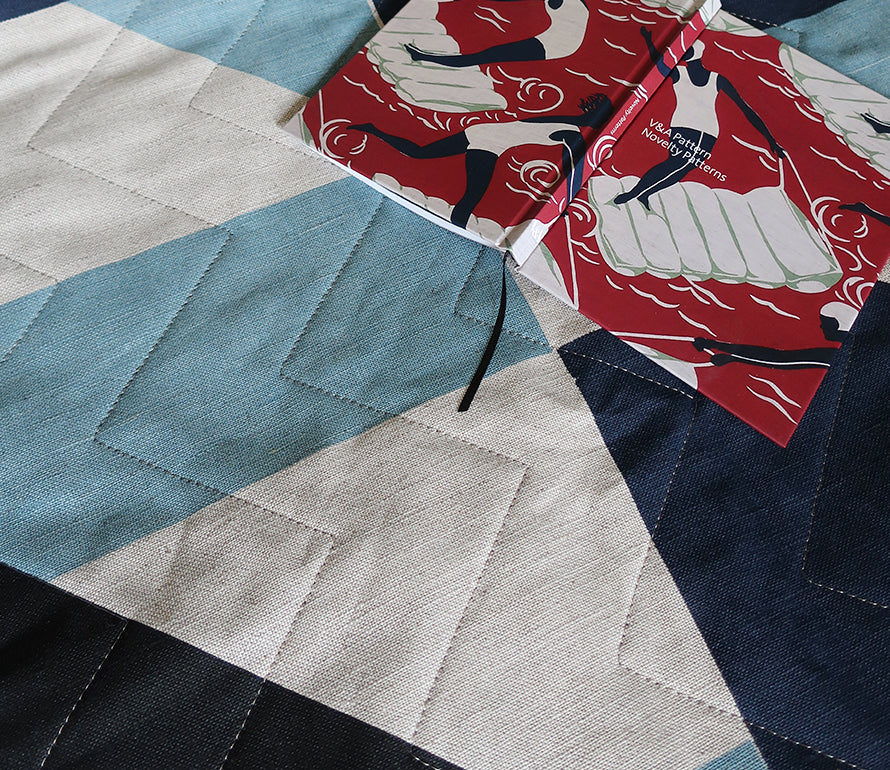The photograph depicts a throw blanket adorned with a vibrant geometric pattern, comprised of various shades of blue, white, khaki, and black. The intricate design features machine-stitched zigzag patterns that run parallel across the fabric, adding texture and dimension to the blanket. Lying face down on this beautifully crafted blanket is an open book titled "V&A Pattern, Novelty Patterns," with the title prominently displayed in white text on its red and white cover. The cover illustration showcases women in vintage swimwear and swim caps, engaging in playful activities on floaty mattresses, with one woman depicted standing and holding a rope at the front of the mattress. The whimsical and nostalgic imagery on the book complements the intricate, handmade appearance of the throw blanket, creating a visually appealing and harmonious scene.